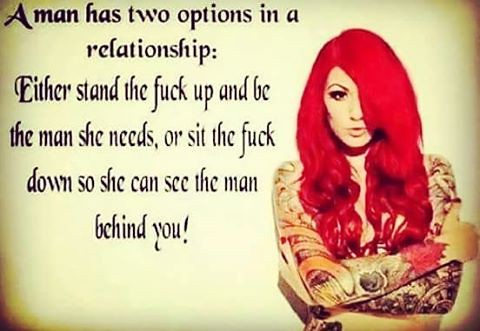The image features a striking card with a bold saying on it. To the right, a woman with captivating red hair, which cascades down to her chest and partially obscures her face, stands with her arms crossed over her chest, showcasing her fully tattooed arms. Her piercing brown eye and arched brown eyebrow give her a defiant look, and her lips are slightly puckered open. She is set against a golden yellow background, with each corner marked by a brown spot. On the left side, the powerful text, written in stylish dark brown to lighter brown fonts, reads: "A man has two options in a relationship: Either stand the fuck up and be the man she needs, or sit the fuck down so she can see the man behind you!" The image uses a color palette of tan, black, red, yellow, and gray, and the overall design seems to convey a message intended for sharing on social media.